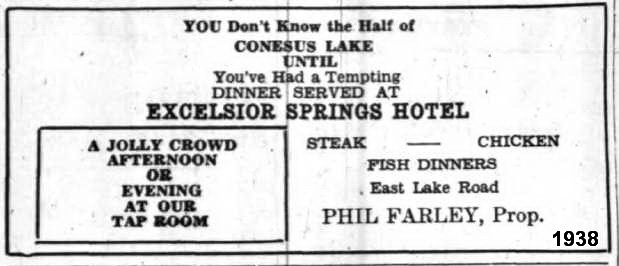This image is a vintage advertisement, designed to resemble an old ticket or newspaper clipping from 1938. The ad is primarily monochromatic, featuring black text on a solid white background with a thin black border, mimicking the shape of a dollar bill. Prominently displayed at the top are the capitalized words, "YOU DON'T KNOW THE HALF OF CONESUS LAKE UNTIL YOU'VE HAD A TEMPTING DINNER SERVED AT EXCELSIOR SPRINGS HOTEL." Just below, a black-outlined rectangle advertises, "A JOLLY CROWD AFTERNOON OR EVENING AT OUR TAPROOM." In the bottom section, the types of dinners are listed: "Steak, chicken, fish dinners." The address "East Lake Road" and "Phil Farley, Prop" (Proprietor) are also included, indicating the location and owner of the hotel. The year "1938" is placed in the bottom right corner, emphasizing the ad's historical context.